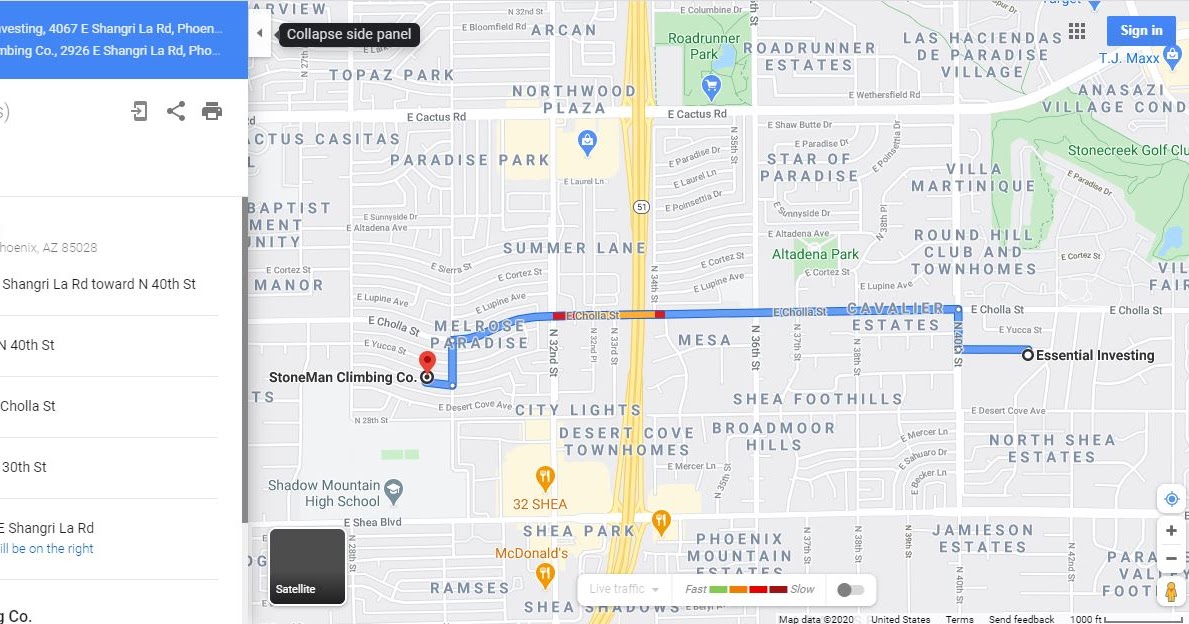This is a detailed screenshot from a maps application. The top portion of the screen features a blue bar displaying the destination address in white text. Just beneath this bar are icons, allowing users to send or print the map. Below these icons lies the route information, with the current directions stating: "Shangri-La Road toward North 40th Street." The majority of the screen is dominated by the map itself, which has a light gray background with numerous detailed roads outlined in white.

A prominent highway, depicted in yellow, runs vertically through the center of the map. A blue route is clearly marked, indicating the path from Stone Man Climbing Company to Essential Investing. This route travels along East Cholla Street. Stone Man Climbing Company is highlighted with a red pin.

In the upper right-hand corner of the map, two parks are indicated by green markings. The names of various towns or neighborhoods are displayed in uppercase gray letters, providing clear geographical context.